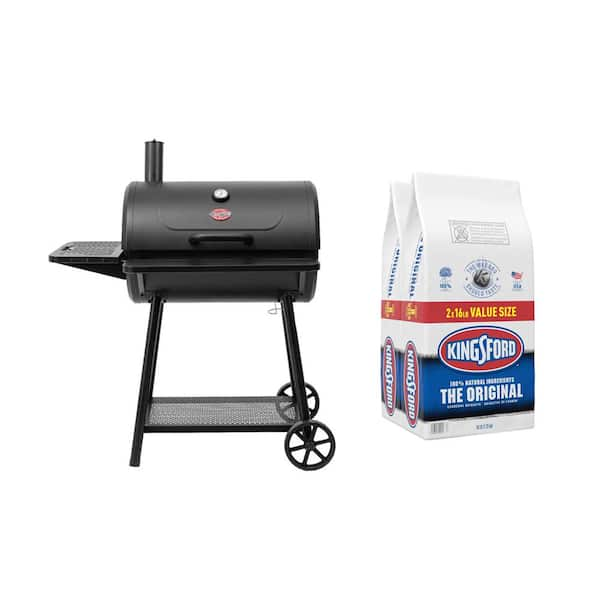The image features a black charcoal grill with a lid that has a handle. The grill is positioned on a metal stand with two solid legs on the left and two wheels on the right, connected by a bottom tray for storage. A small, white dial temperature gauge is visible on the middle of the grill's lid, and a red emblem is located beneath it. On the left side of the grill, there is a side shelf for placing items while cooking. The grill also features a cylindrical vent or spout at the top.

To the right of the grill are two value-sized bags of Kingsford Original Charcoal. The bags are predominantly white with red and blue accents. Each bag displays a red band labeled "value size" across the middle, with an emblem and additional insignia above it. Below the red band, the Kingsford logo is prominently featured in an oval, with "The Original" written beneath it in white letters against a blue background. The image is set against a white background, emphasizing the products.